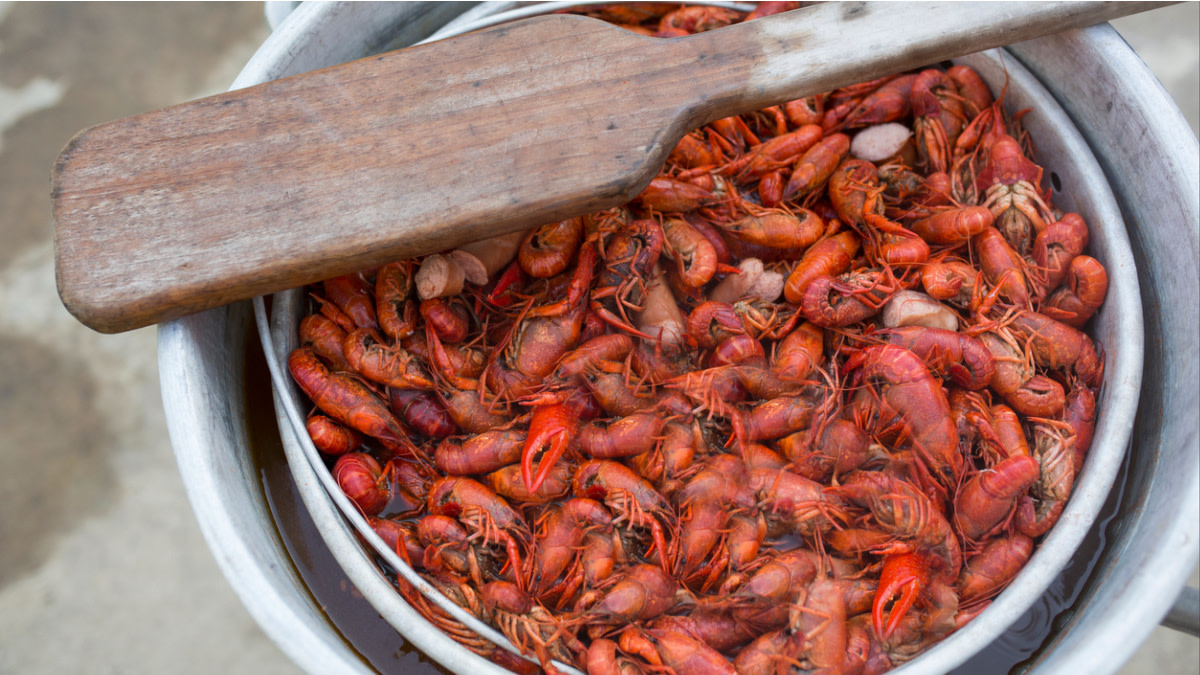In this photograph, there is a detailed scene showing a large white stone-looking bowl that holds a silver bucket. This bucket, possibly of metal, contains a variety of seafood, predominantly red, orange, and clear-colored. The seafood includes what appear to be prawns, lobster claws, and small lobsters, indicated by the presence of tentacles and other distinctive features. The entire setup is on a slightly wet concrete surface. Suspended above the bowl and bucket is a large wooden oar, which is wet at its head and varies in color from light gray to dark brown. This oar likely signifies how the seafood was transported and gives context to the still-life arrangement of the image.